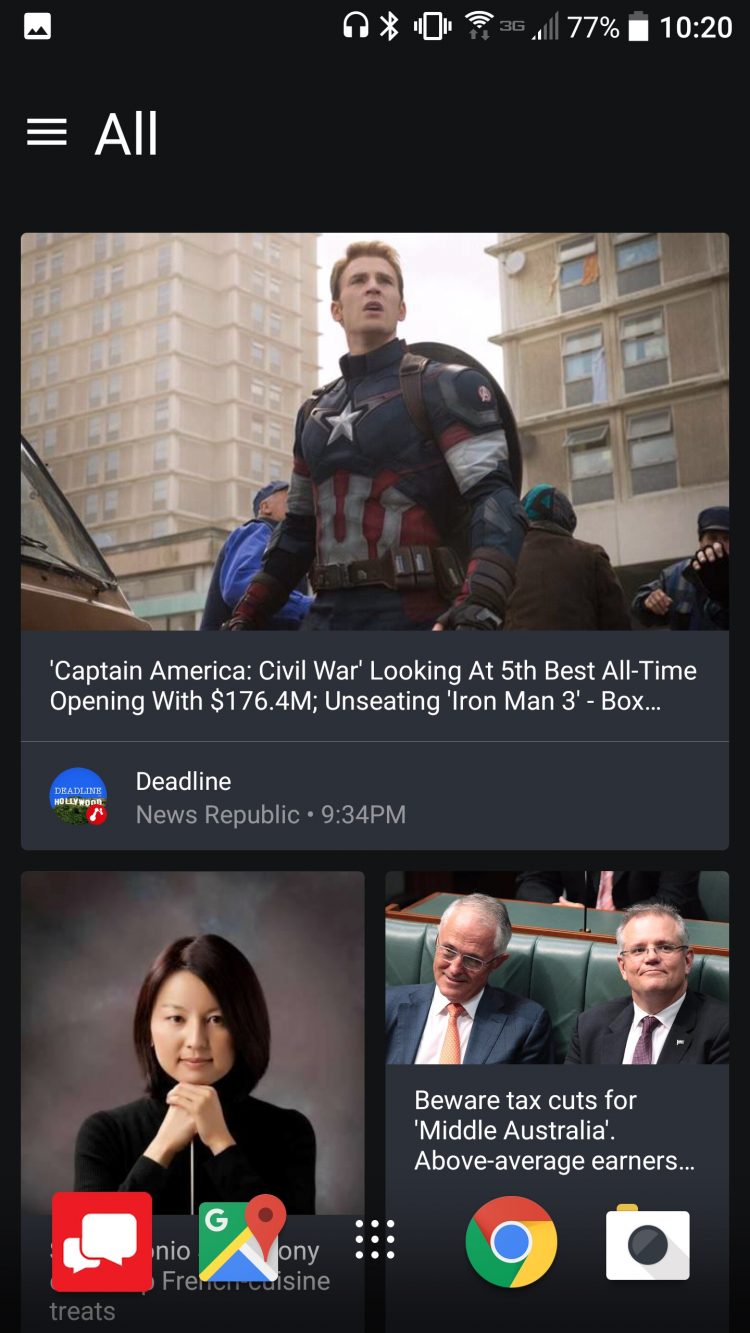The image appears to be a screenshot from a news segment within a mobile app, presumably running on a Google or Android operating system. The interface features a sleek black background with white text, offering a clear and contrasting view of the content. 

At the top, there is an article from News Republic, highlighting a "Deadline" piece about the movie "Captain America: Civil War," focusing on its box office results. Below, two more articles with a business focus are displayed. One features a business-oriented headline with an image of an Asian woman facing the viewer, while the other shows two men in suits with a headline warning about tax cuts for Middle Australia, suggesting the app might be popular or specifically designed for an Australian audience.

At the bottom of the screen, several app icons are visible, including one for a messaging app, Google Maps, Google Chrome, and a camera, indicating the image was captured from a user’s home screen or an app drawer.